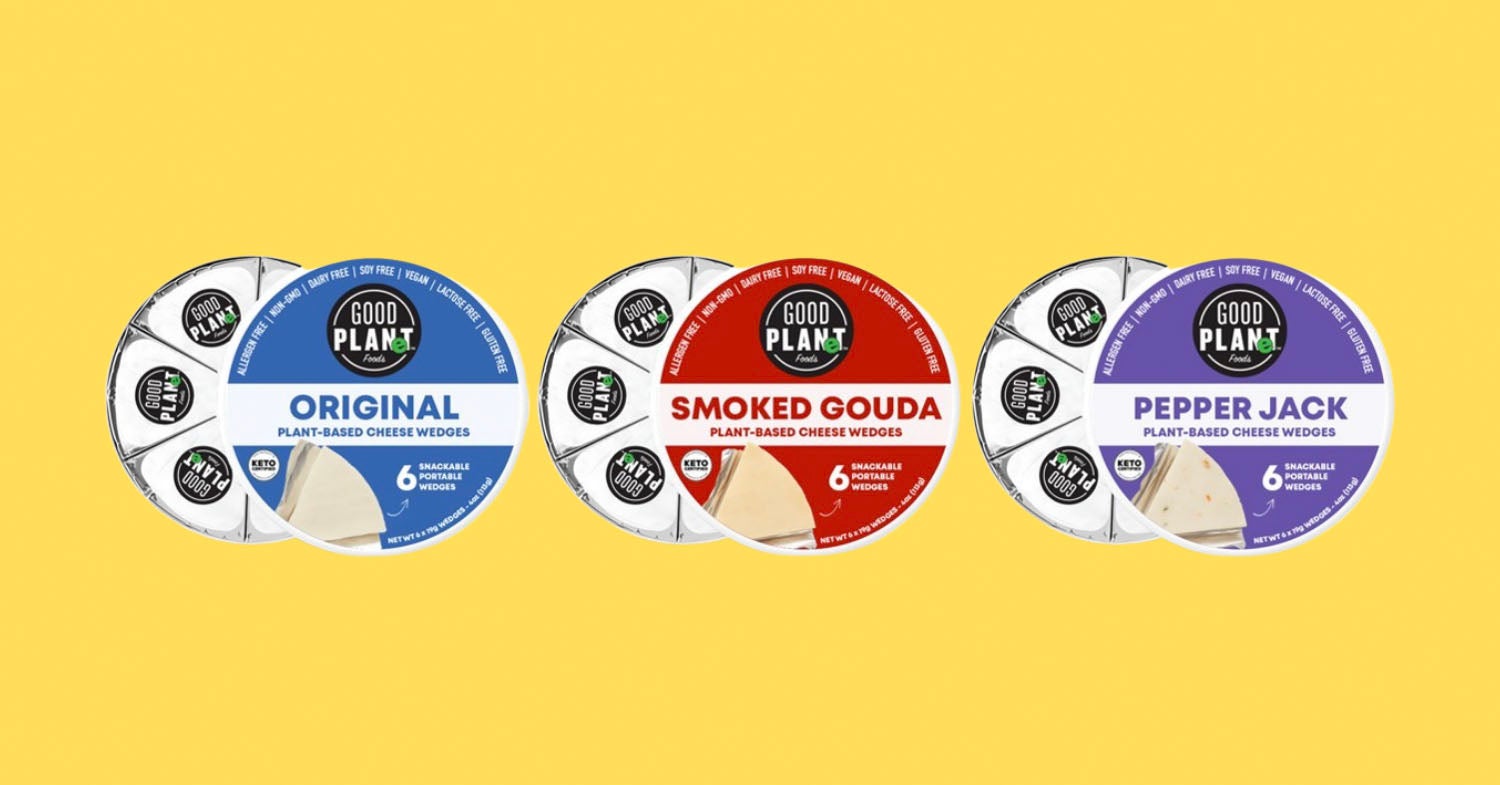The image is a horizontally aligned, rectangular advertisement featuring three different packages of plant-based cheese from the brand Good Planet. The solid dark yellow background accentuates the three circular packages prominently displayed in the center. Each package is a six-pack of individually wrapped triangular cheese wedges. 

- **Left**: The first package, with a blue and white label, is for the original cheese. The top of the label displays the Good Plant brand name, followed by the word "Original" across a white strip in the center. An image of the cheese and the number six are featured at the bottom of the label. This package has three wedges visible, positioned to the left of the partially open cover.

- **Middle**: The second package showcases the Smoked Gouda cheese with a striking red and white label. Just like the original, the Good Plant brand name is at the top, "Smoked Gouda" in red letters across the central white strip, and an image of cheese with the number six at the bottom. Three of its six wedges are similarly displayed to the left.

- **Right**: The third package highlights the Pepper Jack variety with a purple and white label. The Good Plant name again appears at the top, "Pepper Jack" is written in purple across the white strip at the center, and an image of the cheese with the number six is at the bottom. The package is partially opened to reveal three of its six wedges to the left.

The display is meticulously organized, showcasing the neatly aligned labels and partially opened covers to allow a clear view of the triangular cheese wedges, making it an effective advertisement for both online use and store circulars.